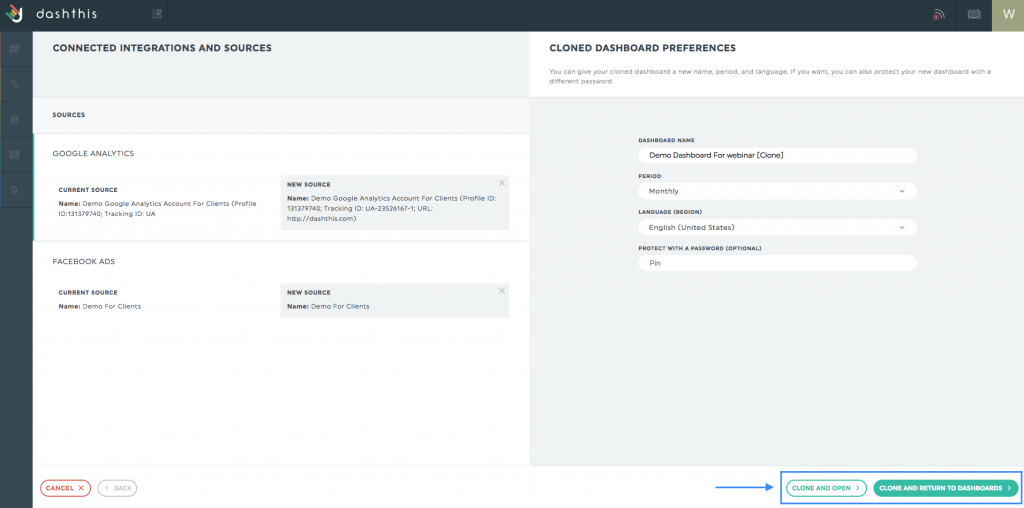The image appears to be a screenshot of a web page interface, predominantly featuring a dark black background encompassing the top and left sides. At the top of the image, the phrase "DashThis" is prominently displayed in a hand-drawn style, resembling a hand making the "I love you" sign in American Sign Language, with the two middle fingers folded down and the pointer and pinky fingers extended upwards. 

To the right side, under faint visibility, there are five clickable icons arranged vertically on the left. At the top center of the interface, the text "Connected Integrations and Sources" is visible. To the top right, options labeled "Cloned Dashboard Preferences" are present.

The interface is punctuated by various clickable elements distributed throughout the image. At the bottom left corner, a red "Cancel" button is located. On the bottom right, two green buttons labeled "Clone and Open" and "Clone and Return to Dashboard" are situated.